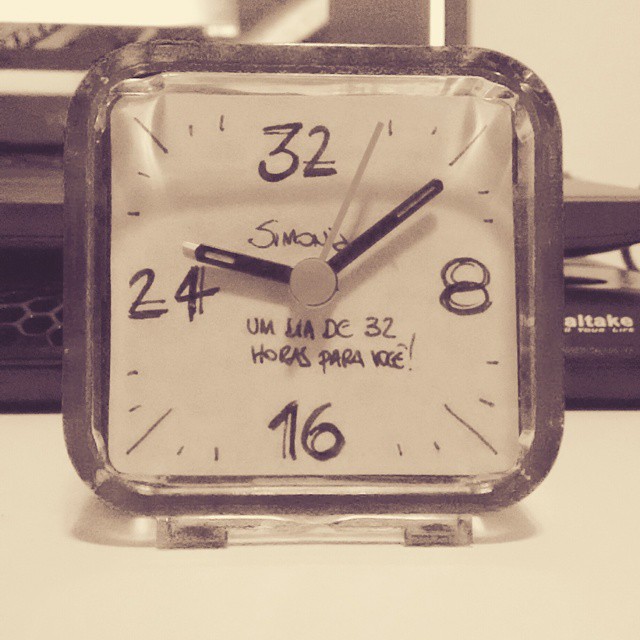The image features a square-shaped clock resting on a light gray tabletop. The clock is prominently zoomed-in, showcasing its dark gray square frame. The clock face displays numbers in an unconventional arrangement: 32 at the top, 8 on the right, 16 at the bottom, and 24 on the left. In between these numbers are several smaller lines and dashes.

The clock hands are black; the shorter hand points to 24, while the longer hand is positioned between 32 and 8. At the bottom of the clock face, Spanish text reads "un dia de 32 horas para voce!" which translates to "a day of 32 hours for you!" 

In the background, a black object is partially visible, adding a touch of contrast to the scene. In the bottom right corner of the clock, the letters "e-i-t-e-k-e" can be seen. The upper right corner of the image also shows a continuation of the light gray color that makes up the tabletop.